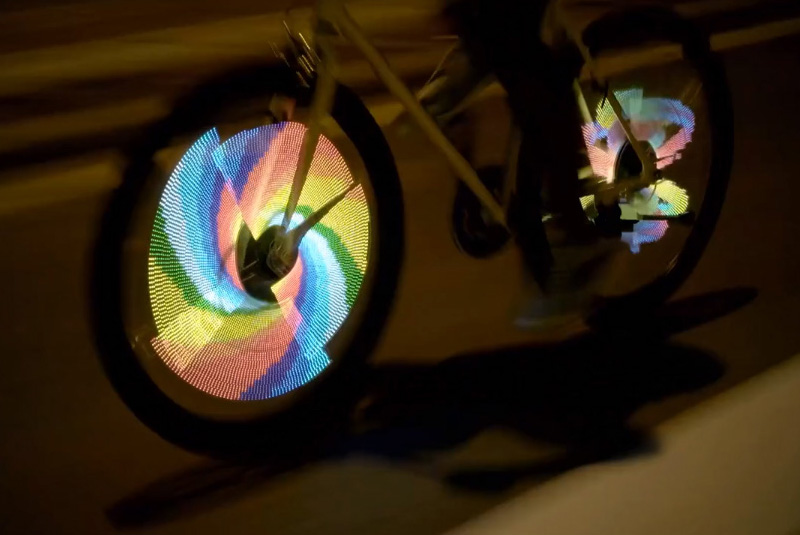This nighttime landscape photo captures the lower half of a bicycle in motion, likely utilizing a long exposure technique to highlight the vibrant, swirling lights attached to its wheels. The front wheel is adorned with a mesmerizing spiral of colors—light blues, dark blues, orange-pinks, yellows, greens, and whites—creating a beautiful, fan-like rainbow effect reminiscent of an atom with swirling electrons. Though the image is blurred, emphasizing the dynamic movement, the brilliant lights on the spokes illuminate both sides of the bike frame, casting colorful reflections into the shadowy background. The rear wheel, partially obscured by the bike’s gears, mirrors the front wheel’s captivating light display, albeit less prominently. The overall effect is both visually striking and artistically rendered, showcasing the stunning interplay of colors against the dark night.